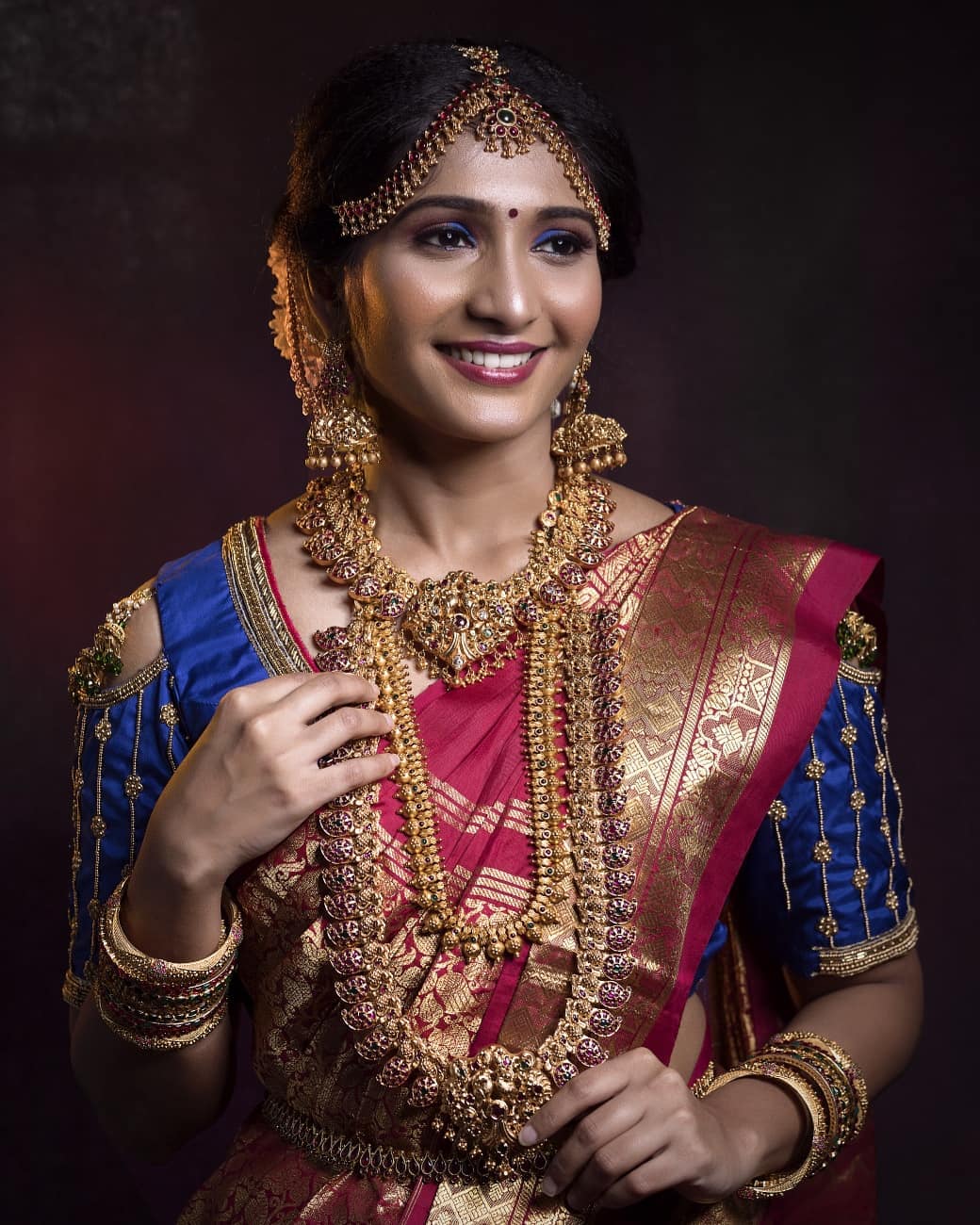This is a professional photograph of a confident South Asian woman, likely of Indian descent, with a warm, broad smile. She is adorned in elaborate, luxurious attire that features a mix of vibrant colors such as gold, blue, red, and burgundy. Her black hair is complemented by a traditional headdress. She has caramel-colored, light tan skin and is wearing an ornate golden necklace, heavy gold earrings, and matching bracelets on both wrists. Her outfit includes a golden vest-like garment with intricate blue threading on the shoulders and additional golden thread accents. The backdrop of the photo is a sophisticated blend of dark red and gray, adding depth and richness to the overall composition.